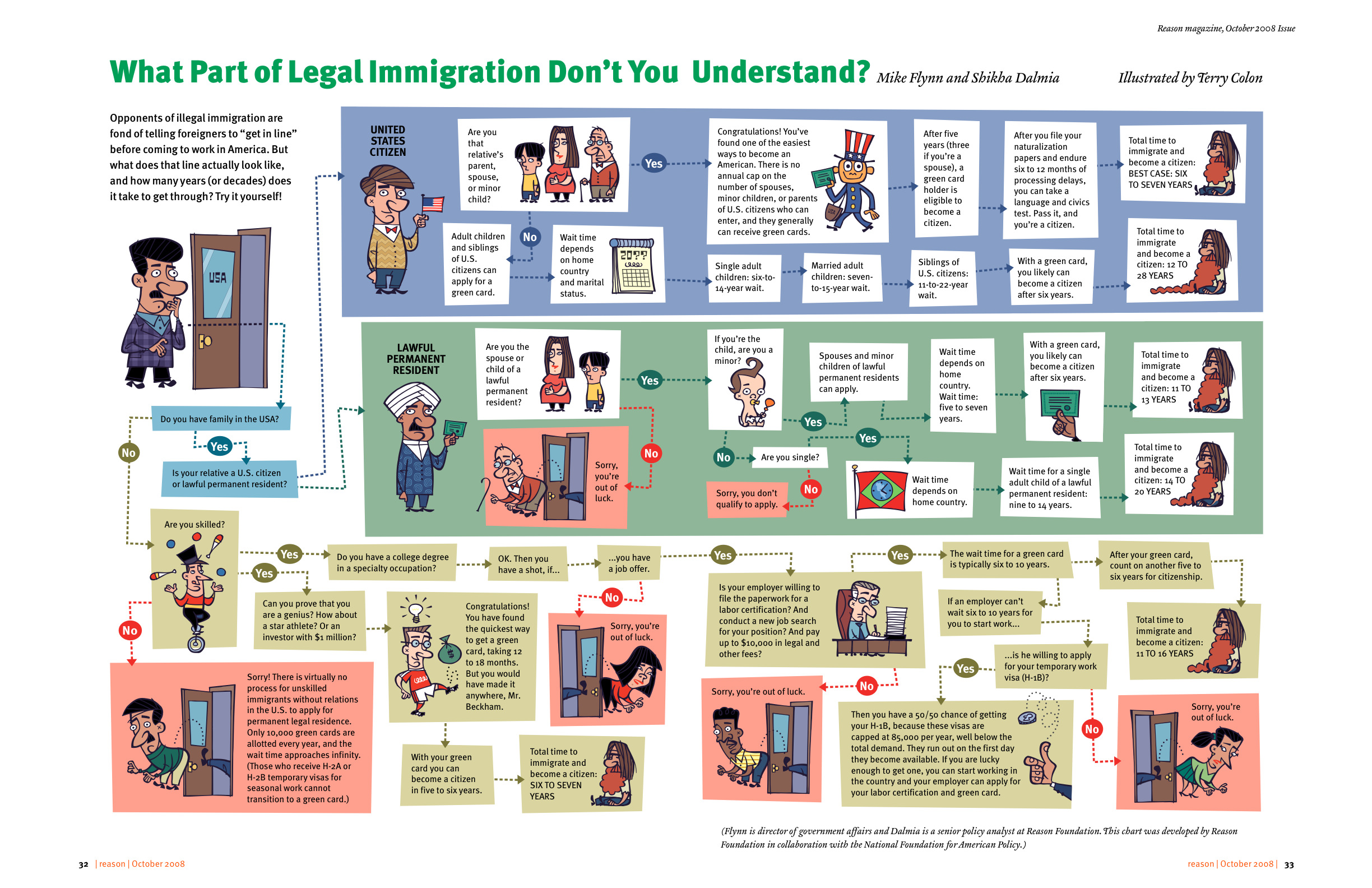This is a detailed description of a poster about legal immigration. 

At the very top of the poster, there is a bold, green heading that reads, "What part of legal immigration don't you understand?" Following this, in a smaller blue font, are the names "Mike Flynn and Shehiba Dalmas," attributed with the phrase "Illustrated by Terry Cohn."

The poster provides an in-depth explanation of the legal immigration process using a series of cartoons and arrows to guide the reader through each step, making the complex process more understandable. The first segment, which is highlighted in a block, states: "Opponents of legal immigration are fond of telling immigrants to 'get in line' before coming to work in America. But what does that line actually look like? And how many years (or decades) does it take to go through? Try it yourself."

Following this initial explanation, the poster leads the reader to the next step with the question, "Do you have family in the USA?" This question branches off into subsequent steps based on the reader's response, detailing different pathways and timelines involved in the legal immigration process. Each step is visually represented with illustrations and directional arrows, but the finer details might be challenging to read due to the complexity and length of the portrayed process.